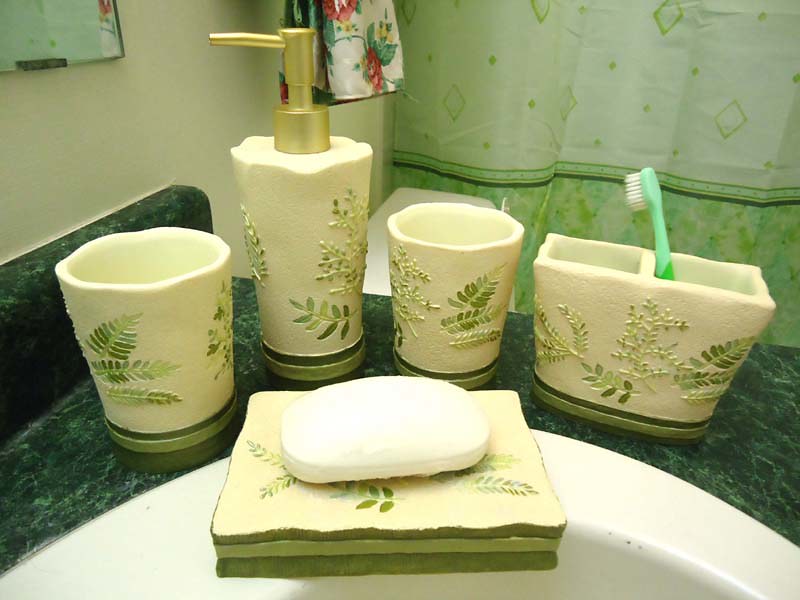The image features a set of five bathroom accessories. In the forefront, there are two bathroom cups, possibly for holding water. A soap dispenser with a golden pump sits among them, exuding elegance. Accompanying these is a toothbrush or toothpaste holder, designed with two compartments for enhanced convenience. A soap dish, featuring a bar of soap, completes the ensemble. These items exhibit a creamy white color adorned with green leaf patterns, giving them a natural aesthetic. They appear robust and durable due to their thick construction. In the background, the top edge of a toilet and a green shower curtain are visible, with a partial glimpse of a mirror in the top left corner, framing the setting of a well-coordinated bathroom.